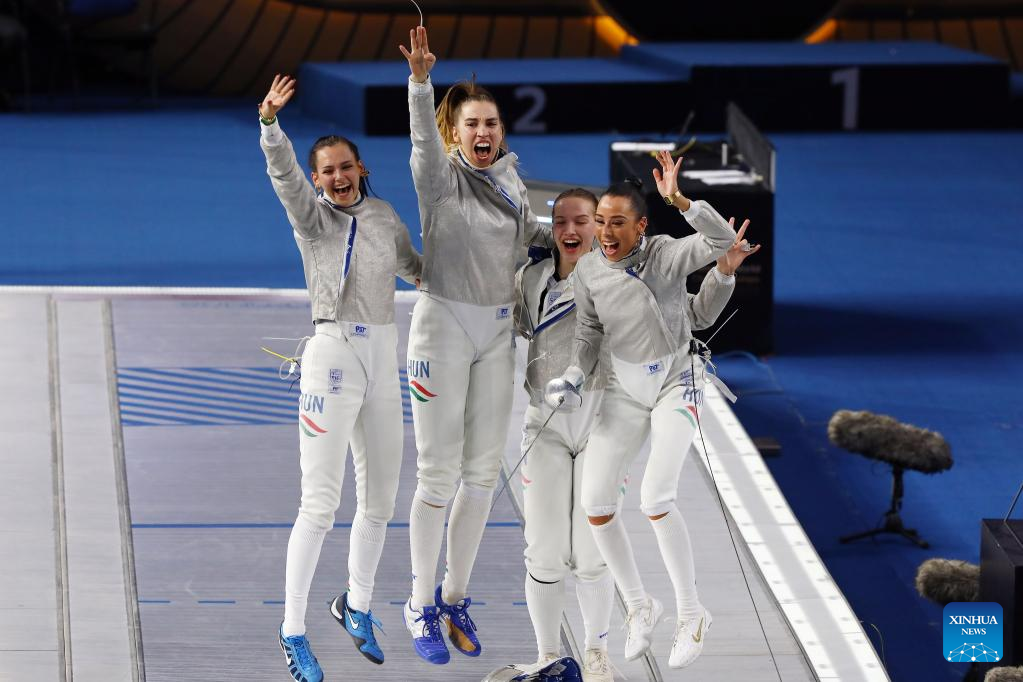This photograph captures the jubilant celebration of four young female fencers who appear to be part of the Hungarian Olympic team, as indicated by the "H-U-N" lettering and the red, white, and green flag on their white pants. They are energetically leaping in the air, expressing their joy after a triumphant win, possibly at the Olympics. Three of them are mid-air while one remains on the ground, all displaying exuberant smiles. Their uniform consists of white pants, grey jackets, and blue and white shoes. Some of the fencers are still holding their épées. Behind them, an empty podium with designations for first and second place can be seen, alongside a blue backdrop set up for medal presentations, which also shows the logo "Xinhua News" in the bottom right-hand corner. The scene is vibrant and captures a moment of pure elation and pride.